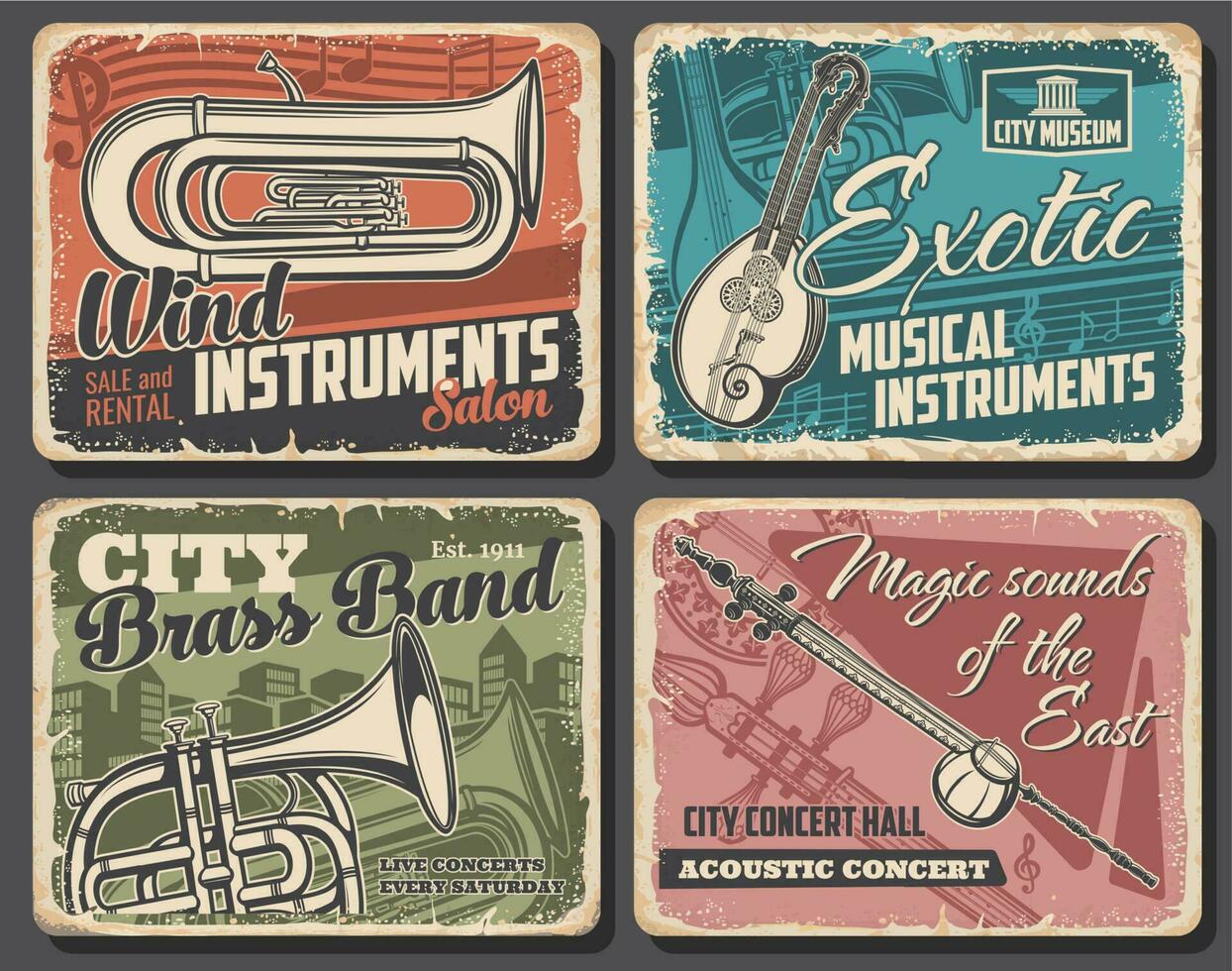The rectangular image, wider than it is tall, features a dark gray background adorned with four colorful, credit card-shaped sections, one in each corner, each advertising various music-related events or services. 

In the top left section, which has an orange background with musical prints, the text reads "Wind Instruments, Sale and Rental Salon," accompanied by an off-white illustration of what appears to be a tuba, marked by its coiled middle section. A brownish-gray border decorates the bottom.

The top right section, set against a medium blue backdrop, showcases the words "City Museum, Exotic Musical Instruments" in white. It features an image of a unique, double-handled string instrument that seems to be a sitar or an unusually designed guitar.

In the bottom left section, with an army green two-tone background, the text "City Brass Band, Established 1911" stands out in white and black. It displays another brass wind instrument, possibly a French horn, and notes "Live concerts every Saturday."

Lastly, the bottom right section, primarily pink with a darker red hue, highlights "Magic Sounds of the East, City Concert Hall" in white text, and "Acoustic Concert" written in a black band at the bottom. It features a black and white depiction of a long, flute-like instrument with an extra round piece in the middle.

Each section vividly represents a distinct musical theme, contributing to a vibrant and engaging overall composition.